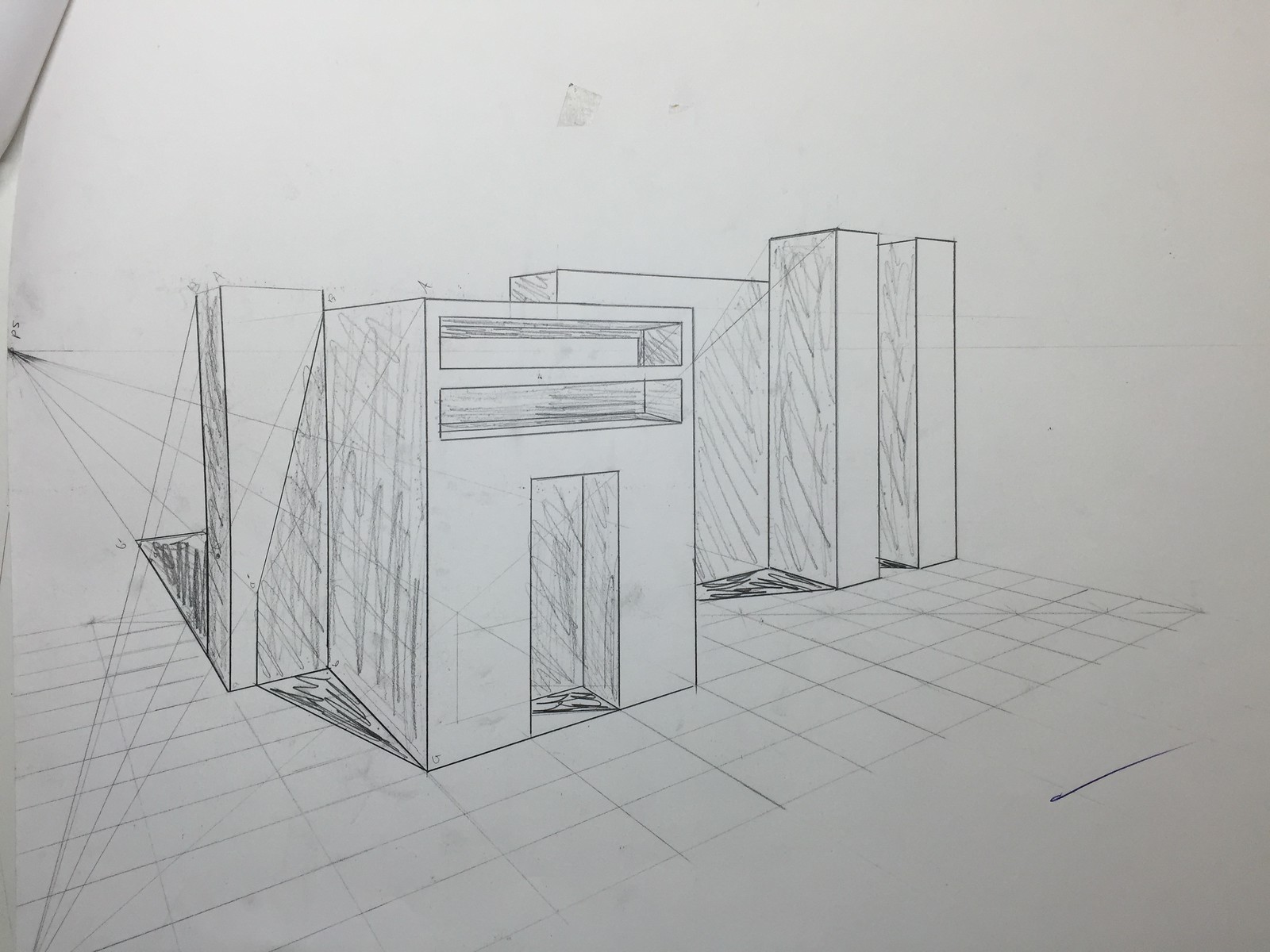A meticulously detailed pencil or charcoal drawing on a white background showcases a checkered floor composed of presumably tiled squares. Dominating the scene are five upright, cuboid structures with various recesses carved into their solid forms, suggesting they might be constructed from concrete. The objects, varying in height, display intricate shading on their left-hand sides, providing depth and definition to the composition. The artist's technique skillfully captures the textures and dimensionality of both the floor and the solid geometric figures, creating a striking visual contrast.